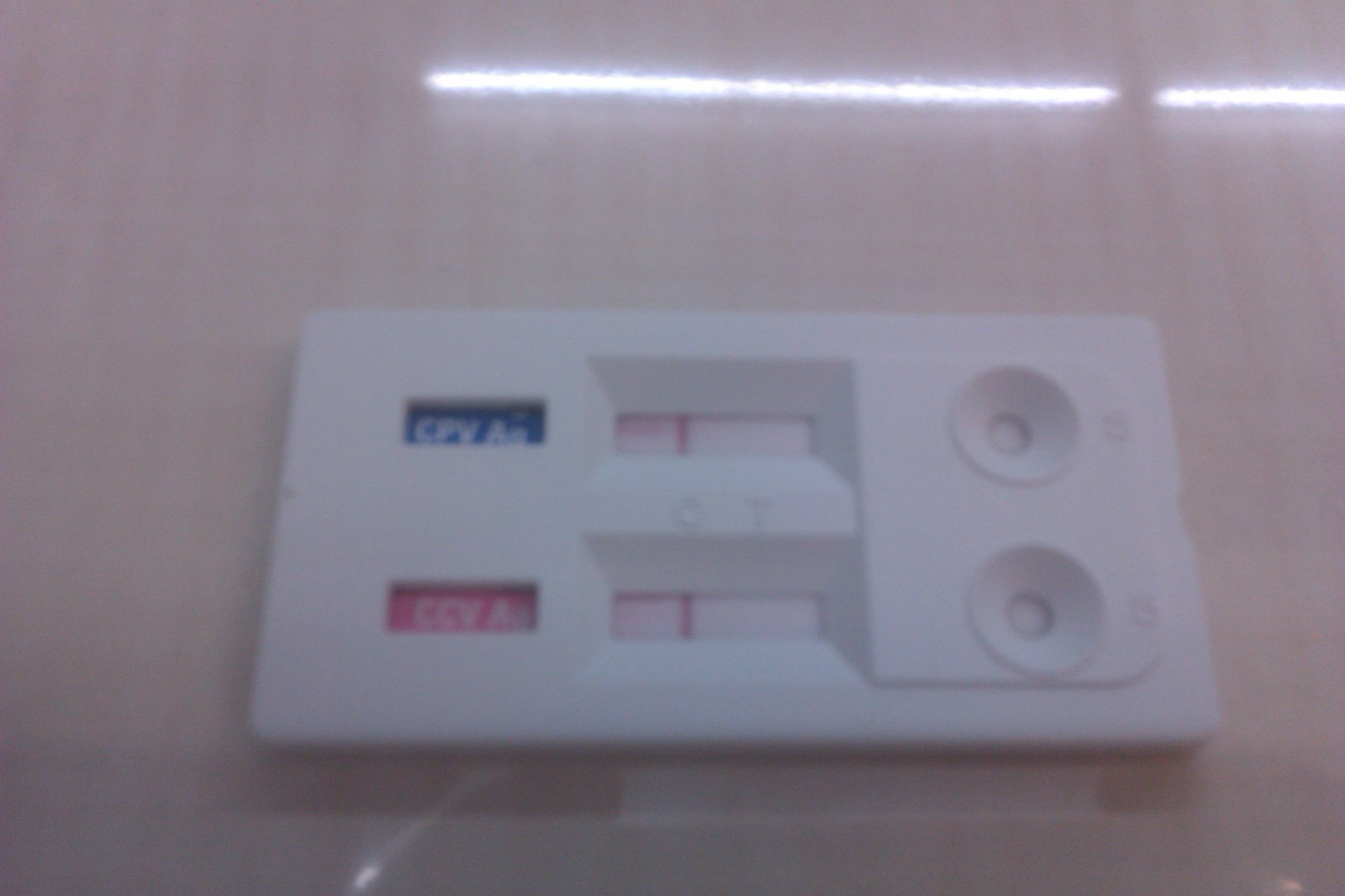This is a photograph of a white, wall-mounted device featuring a complex interface. It has two small rectangular windows positioned one above the other. To the right of these windows are two recessed, round sections whose purpose is unclear. Adjacent to these sections, possibly on the left side, there are two displays aligned vertically. 

The top display is a smaller rectangular window with a blue background that shows white letters spelling out "CPA." Below it, a larger display features red letters on a white background, spelling "CCVA" or something similar. The entire device appears to be made of plastic and is affixed to a shiny wall, which also seems to be plastic.

In the reflection on the wall, two long fluorescent lights on the ceiling are visible, indicating the setting is well-lit. The overall appearance suggests a control panel or monitoring device in a clean, well-maintained environment.